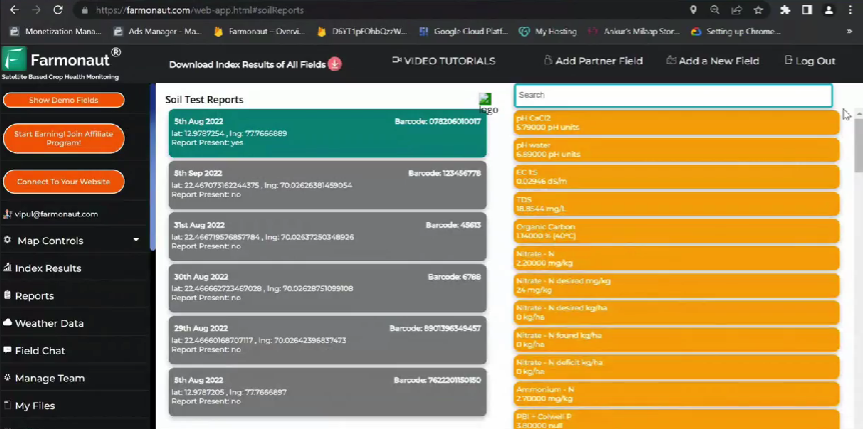The image features a user interface with a black background. At the top of the screen, there is a green box on the left side, displaying a Japanese character resembling 'F'. Adjacent to it, text reads, "Pharma," alongside options including "Download Index," "Results of All Fields," "Video Tutorials," "Add a Partner Field," "Add a New Field," and "Log Out."

On the left-hand side, there are three reddish-orange buttons labeled "Show Demo Fields," "Start Earning through Affiliate Programs," and "Connect to Your Website." Towards the bottom of this section, additional options are listed such as "Maps," "Index Reports," "Weather Data."

In the center of the interface, there are two columns related to "Soil Test Reports," presenting six report choices. Fields include terms like "pH," "Co," "C12," "pH Water," "Organic Cation," and other organic measurements, intended to assist farmers.

The text elements throughout the interface are primarily in tangerine orange, enhancing visibility and aesthetics. Some sections are blurred, but the essential details focus on providing useful agricultural data for farmers.